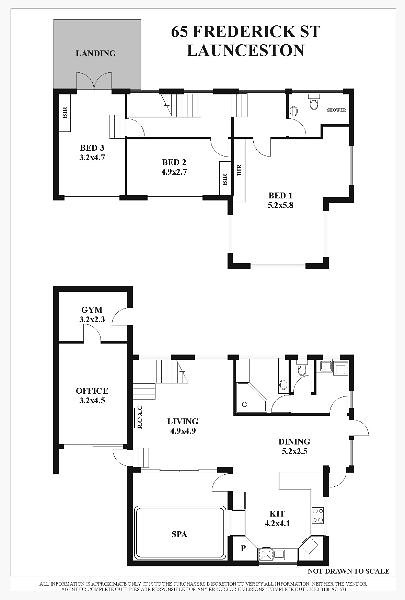This image features a detailed black-and-white floor plan for a house located at 65 Frederick Street, Launceston. The plan is depicted on a white sheet of paper with black text and illustrations clearly delineating the layout of two separate floors.

The first floor plan, situated on the upper portion of the image, includes three bedrooms labeled as Bed 1, Bed 2, and Bed 3, with each room's dimensions provided. Notably, Bedroom 3 has doors leading to a landing area.

Below the first plan, the second floor plan illustrates various living spaces including a living room, dining area, office, gym, and spa, each accompanied by their corresponding dimensions.

A note at the bottom of the image specifies that the plans are not drawn to scale. Additionally, there is some text at the very bottom, though it's too small and blurred to discern, likely indicating the source of the drawing. Overall, the image serves as a straightforward, yet informative, representation of the floor plans for the property at 65 Frederick Street, Launceston.